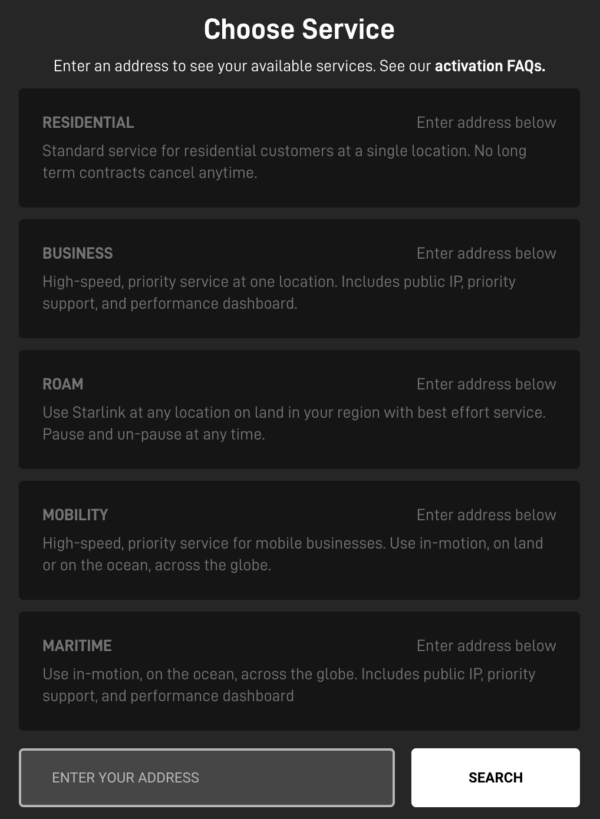This is a screenshot of an internet service selection interface. The image is vertically oriented, with a dark background that appears to be a shade of grayish-black. At the top center, large white text reads "Choose Service." Beneath this, smaller white text instructs users to "Enter an e and address to see your available services. See our activation FAQs," with "Activation FAQs" in bold white font, indicating it is likely a clickable link.

Below these instructions are five wide rectangles with darker black backgrounds and gray fonts, each representing different service options. The first rectangle is labeled "Residential," described as "Standard service for residential customers at a single location. No long-term contracts. Cancel any time." To the right of this description, it says "Enter address below," a note that is repeated for all service options.

The subsequent rectangles list the following services:
1. **Business**
2. **Roam**
3. **Mobility**
4. **Maritime**
Each service option has its description and the note about entering an address.

At the bottom of the interface, there's a gray input box with a light gray border labeled "Enter your address." To its right is a corresponding search button in another rectangle, featuring black font and aligned with the address input box. The streamlined design directs users to input their address and search for available internet services based on their choice.